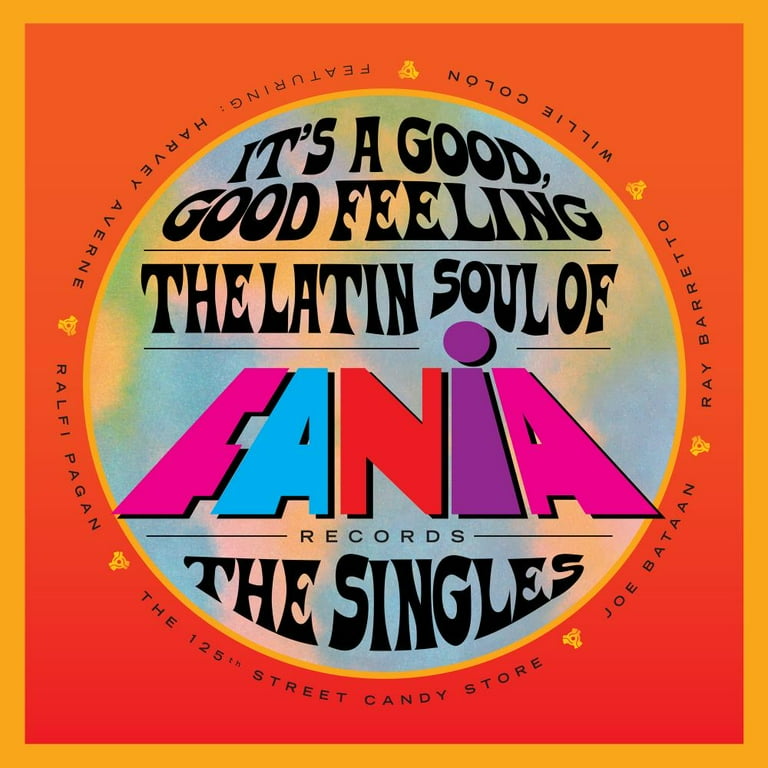The image is a full-color square print piece with a prominent orange border encasing a reddish background. The centerpiece is a large circle occupying most of the image, featuring a hazy bluish-green backdrop. At the top in bold black text, it reads "It's a good, good feeling," followed by "The Latin soul of" in a similar style. Below, in colorful letters, it showcases "Fania," where the 'F' is pink, the 'A' is blue, the 'N' is red, the lowercase 'i' is purple, and the final 'A' is pink. Below "Fania," in large black letters, it states "Records" and "The Singles." Surrounding the central circle are names in black text interspersed with yellow triangular accents: Joe Bataan, Ray Barretto, Willie Colon, featuring Harvey Averne, Ralphie Pagan, and the 125th Street Candy Store. The entire design evokes a nostalgic feel of an album or record cover from a bygone era, emphasizing its rich Latin soul heritage.